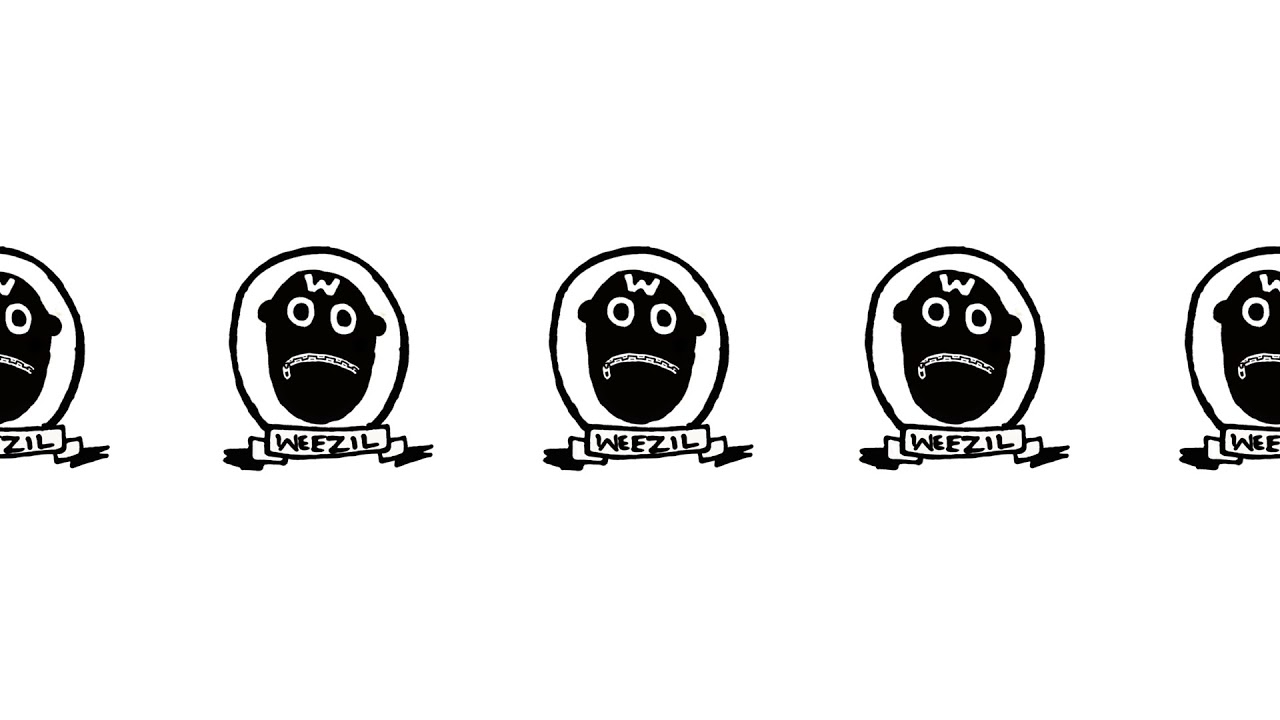The image is a rectangular, digital design with a white background, showcasing a series of identical faces arranged in a horizontal row just below the center. Each face is encased in a blue, oval-like circle outlined in black. The faces are black with distinctive features: a white 'W' on the forehead, white eyes with large black pupils, and a white mouth designed as a closed zipper. The face lacks a nose and has two small ears positioned close to the eyes. Beneath each face, there is a ribbon-like banner in black, with the word "W-E-E-Z-I-L" inscribed in black letters. The row of faces extends across the center, with the outermost faces on the left and right edges only partially visible. The combined elements create a repetitive, eye-catching pattern, emphasizing the quirky, stylized facial design.